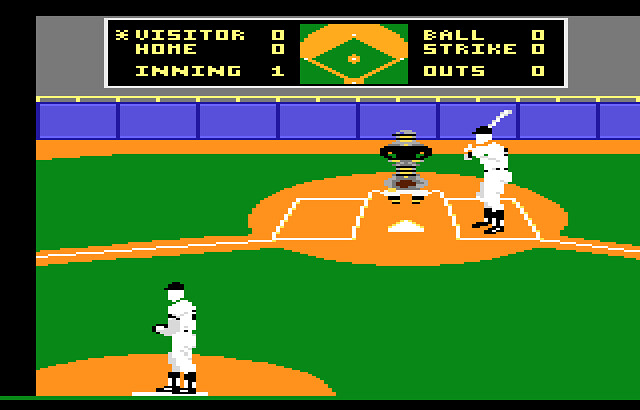The image depicts a nostalgic, pixelated baseball video game reminiscent of the 1980s, possibly an Atari or Intellivision title. The graphics are rudimentary but iconic. In the scene, a batter, dressed in a white uniform with a black cap, stands at home plate holding a white bat. Behind the batter sits the catcher, outfitted in a black, yellow, and gray uniform. The pitcher, located in the lower-left corner, appears in black and white with a black cap, poised to throw. The green field extends in the background, framed by a simple blue backstop.

Above the playing field, the scoreboard displays the game's status in pale yellow text on a black background, bordered by white. The scoreboard reads "Visitor 0, Home 0" with the game in the first inning. Additional stats on the right show "Ball 0, Strike 0, Outs 0." In the center of the scoreboard, a smaller depiction of the baseball diamond is visible, providing an inset view of the field. The overall scene captures the essence of early baseball video games, emphasizing minimalist detail and design.